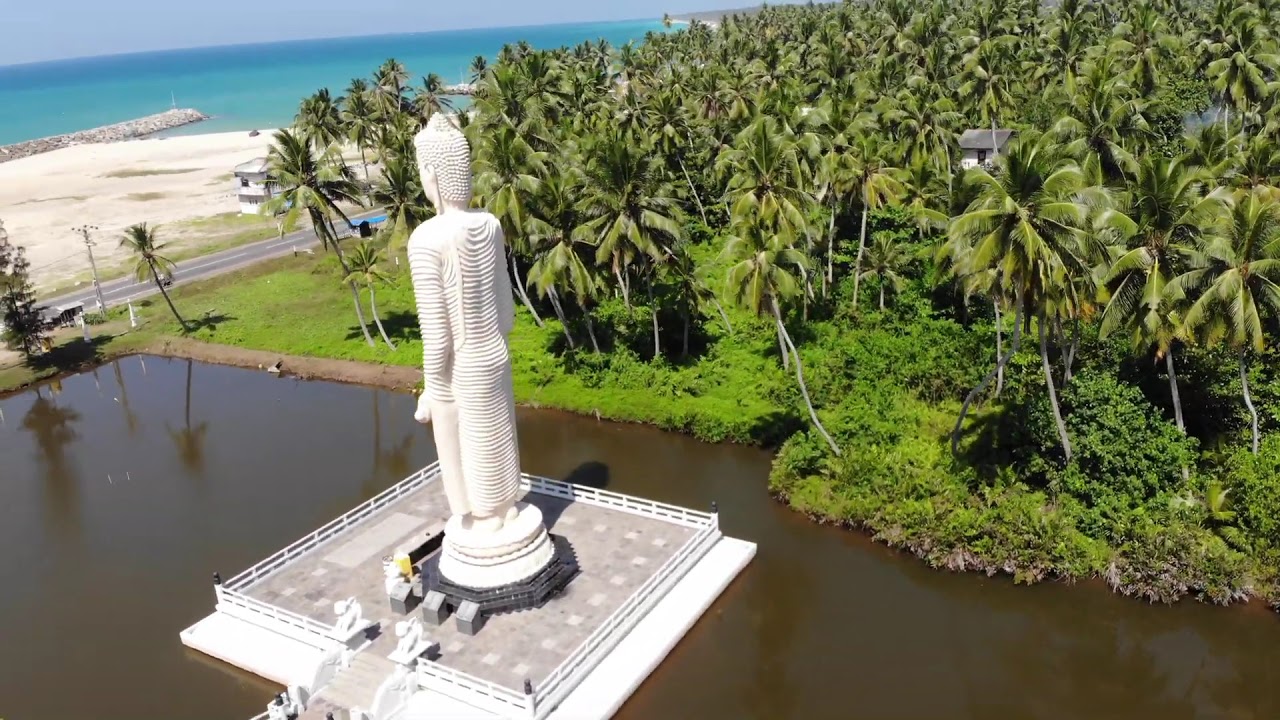This aerial image, captured in a landscape orientation, showcases a scenic coastal area blending natural and architectural beauty. At the center of the image is a large, tall white statue of a Hindu goddess, elegantly draped in traditional attire. The statue is mounted on a white, stone square platform surrounded by a pond of brownish water.

The statue, facing towards the aqua-blue ocean, towers over a dense forest of palm trees, which occupy the background, stretching across the upper right to nearly the lower right corner of the image. The trees contrast strikingly with the blue sky above, creating a lush, tropical ambiance.

In the upper left part of the photograph, a pristine white sandy beach meets the deepening hues of the ocean, interrupted by a rock jetty extending into the water. Separating the pond and statue area from the beach is a road that runs from the middle left towards the middle of the frame, lined with an occasional electrical pole, further enhancing the sense of scale of the imposing statue.

Overall, this drone photograph captures both the grandeur of the statue and the serene beauty of its tropical surroundings, with the clear blue ocean completing the picturesque scene.